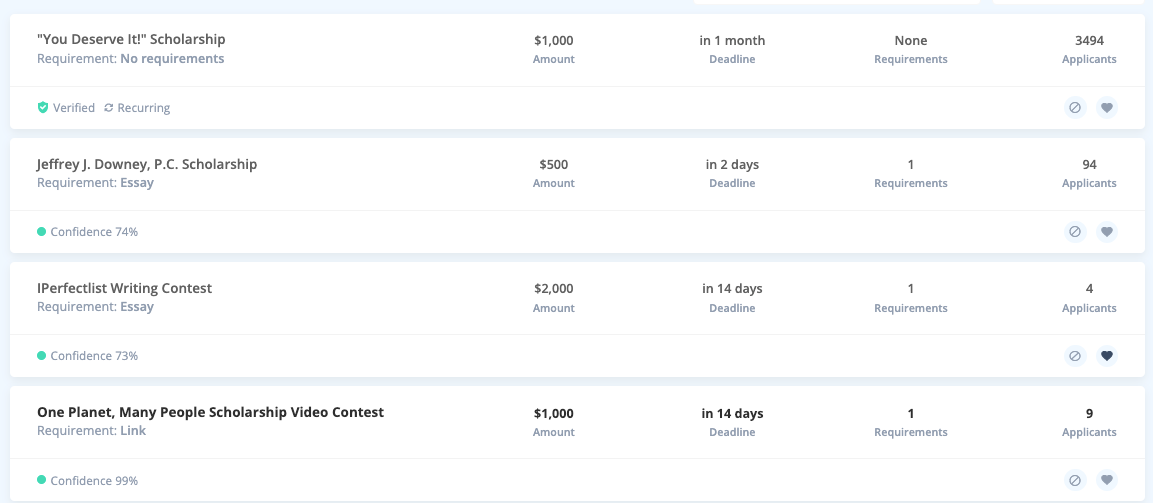The image features a webpage organized with a light blue border, approximately a quarter of an inch thick, that frames the top, left, and right edges. The main content is structured into four horizontal white rectangles, each about two inches in height, that span the width of the page, except for the blue border on the sides. These rectangles are separated by thin blue dividers.

The first section, on the left side, displays scholarship names and details in a stacked format. The top entry reads "You Deserve It" in parentheses, written in black, followed by "Scholarship." Underneath, in smaller black text, it states "No requirements." Below this is a small blue circle with a white checkmark indicating "Verified," followed by "Reoccurring." Similar information is listed for three more scholarships:
1. "Jeffrey J. Downing PC Scholarship"
2. "I Perfect This Writing Contest"
3. "One Planet Many People Scholarship Video Contest"

To the right of the scholarship names, there is a column indicating the scholarship amounts:
1. $1,000 for "You Deserve It"
2. $500 for "Jeffrey J. Downing PC Scholarship"
3. $2,000 for "I Perfect This Writing Contest"
4. $1,000 for "One Planet Many People Scholarship Video Contest"

The next column outlines the application deadlines:
1. One month for "You Deserve It"
2. Two days for "Jeffrey J. Downing PC Scholarship"
3. Fourteen days for "I Perfect This Writing Contest"
4. No deadline for "One Planet Many People Scholarship Video Contest"

Following the deadlines, the next column lists the requirements:
1. None for "You Deserve It"
2. One requirement for "Jeffrey J. Downing PC Scholarship"
3. One requirement for "I Perfect This Writing Contest"
4. One requirement for "One Planet Many People Scholarship Video Contest"

Finally, the far-right column displays the number of applicants:
1. 3,494 for "You Deserve It"
2. A circle with a line through it (indicating perhaps no data or no applicants)
3. A heart symbol to the right of the no-data indicator (possibly indicating a favorite or popular status)

The layout provides a clear and concise summary of multiple scholarships, highlighting key details such as names, amounts, deadlines, requirements, and applicant numbers.